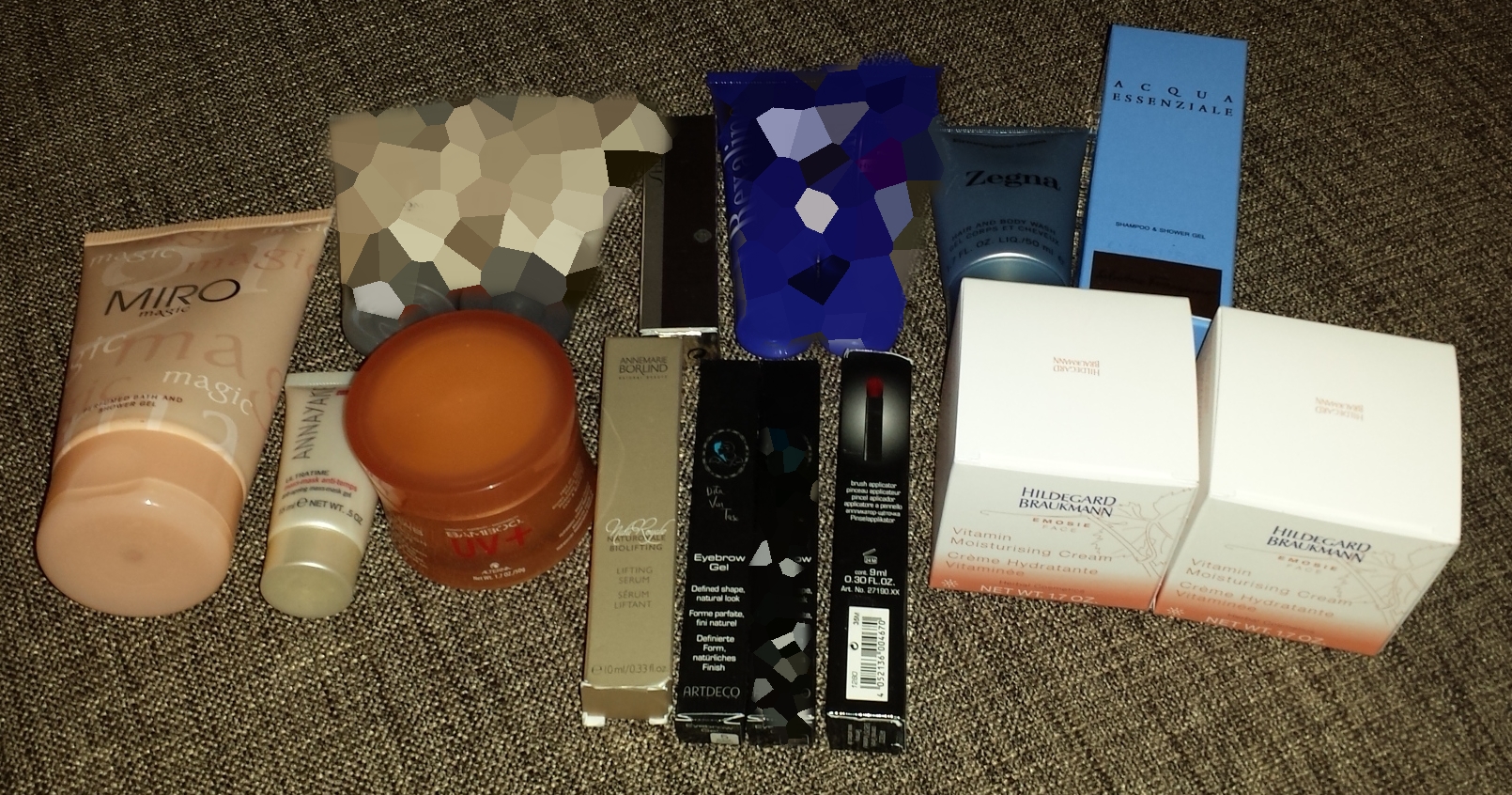A captivating array of cosmetic beauty products is artfully arranged on what appears to be the textured fabric of a sofa, possibly a sofa chair. The collection is a vibrant palette featuring various colors such as skin-tones, white, orange, blue, purple, black, and gold. On the far left, a cream-colored packaging stands prominently labeled "Myro," while adjacent to it, a smaller tube with "ANNAYA" written on it catches the eye despite the remaining text being difficult to decipher. On the far right, a box with the brand name "HILDGARD BROCKMAN" is easily visible; two identical white boxes containing the cream sit beside it. Toward the back, two items are blurred out, adding a touch of mystery to the scene. The assortment seems to comprise creams, and possibly mascara or lipstick, creating a rich tableau of beauty essentials.